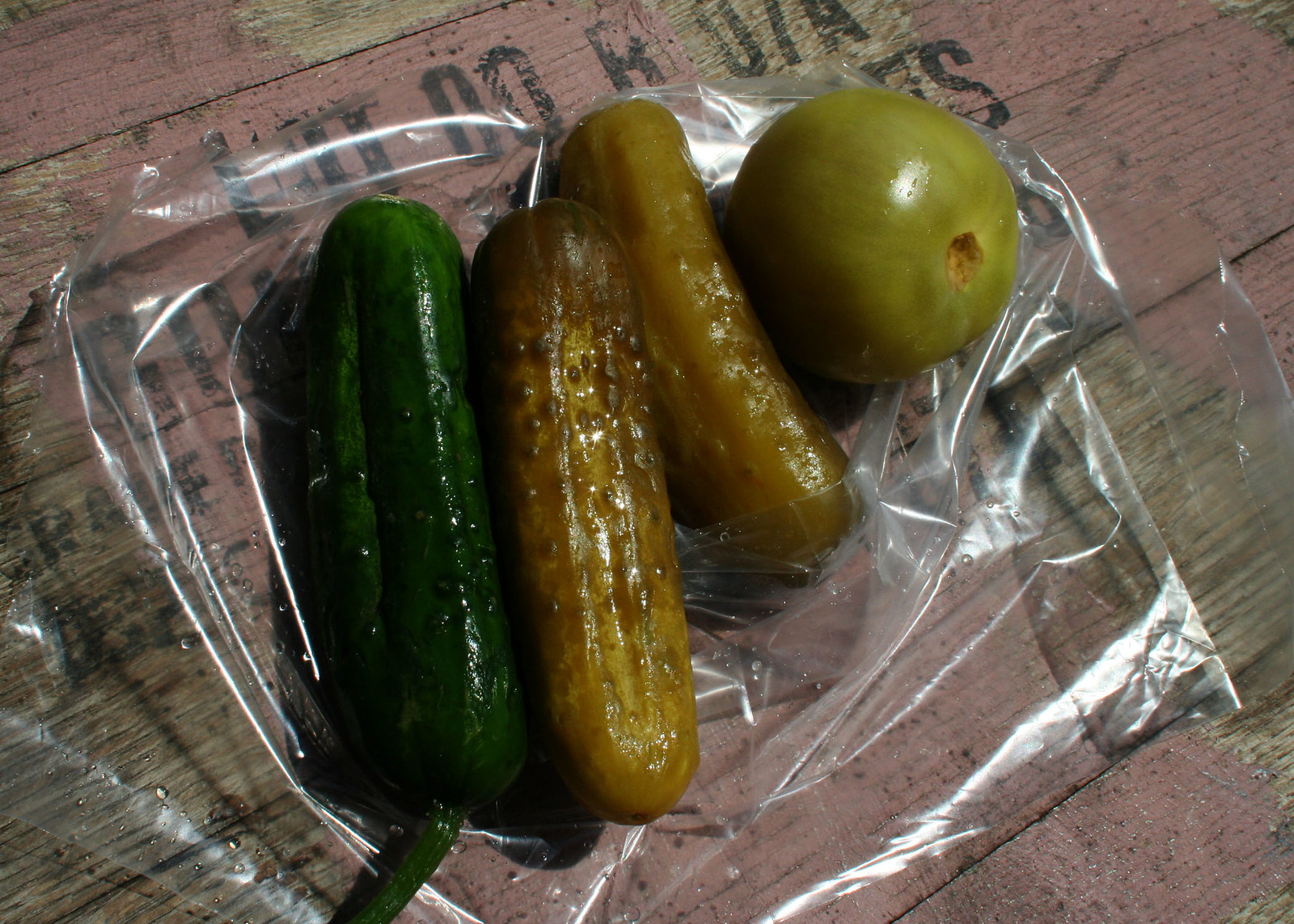In the photograph, several food items — specifically pickles — are carefully arranged on a piece of thick, clear plastic, resembling cellophane. This plastic is placed on a reddish, painted wooden surface, which appears weathered with peeling paint, revealing the wood underneath. The surface probably belongs to a chest, marked with faint, black text etched or painted into it, though the letters are hard to decipher.

The food items centered in the image consist of three pickles and a round green produce item, either a green tomato or a tomatillo. On the left is a bright green pickle, similar in color to a fresh cucumber. In the middle are two larger pickles of a more muted, olive green or brownish hue, indicating they might be treated or boiled. To the right of these pickles is a smaller pickle positioned partially upwards, and finally, on the far right lies the round green produce. The pickles on the left appear slightly wet, while the item on the right does not.